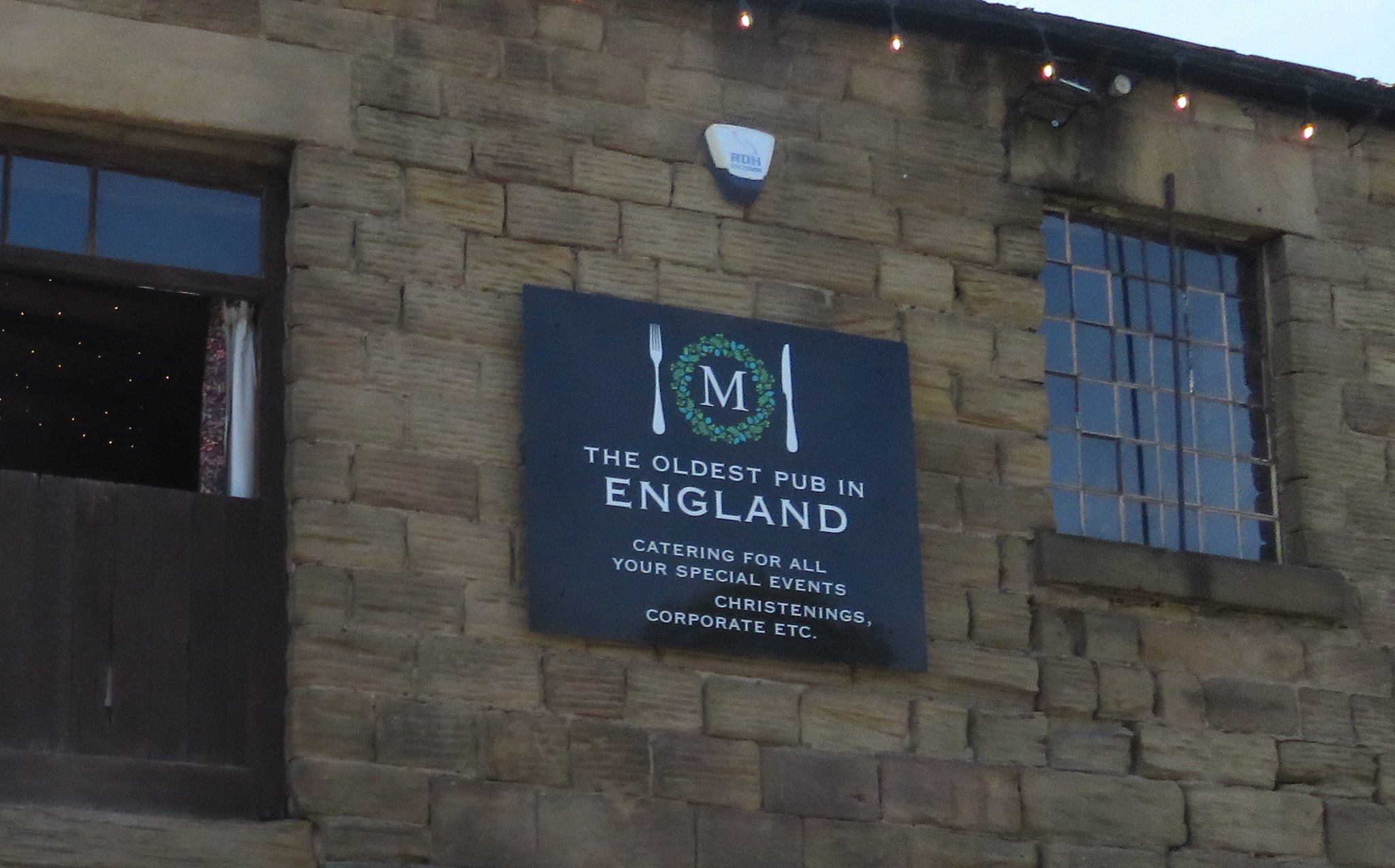The outdoor daytime photograph unveils part of a historic stone building, captured in a rectangular frame that is wider than it is tall. The gray stone facade exhibits a mix of rectangular and square stones, with some appearing patchwork. On the left side, a long stone overhang extends above a feature that resembles a large wooden door, which sports windows at the top and has an open space with a curtain, followed by vertical wooden panels.

Towards the center of the image is a prominent black square sign. This sign displays a logo featuring a white letter "M" encircled by a green wreath, flanked by a fork on the left and a knife on the right. Below the logo, white text announces, "The Oldest Pub in England, catering for all your special events, christenings, corporate, etc." Above this sign, there is a small white device with a blue base, likely an alarm.

To the right of the sign, an old window with metal grid bars adorns the wall, while the top-right corner of the image reveals a sliver of a cloudy sky and the edge of the roof, from which lights are hung. This rich, historical setting is further accentuated by the intricate stonework and the timeless feel of the wooden and metallic elements integrated into the building's structure.